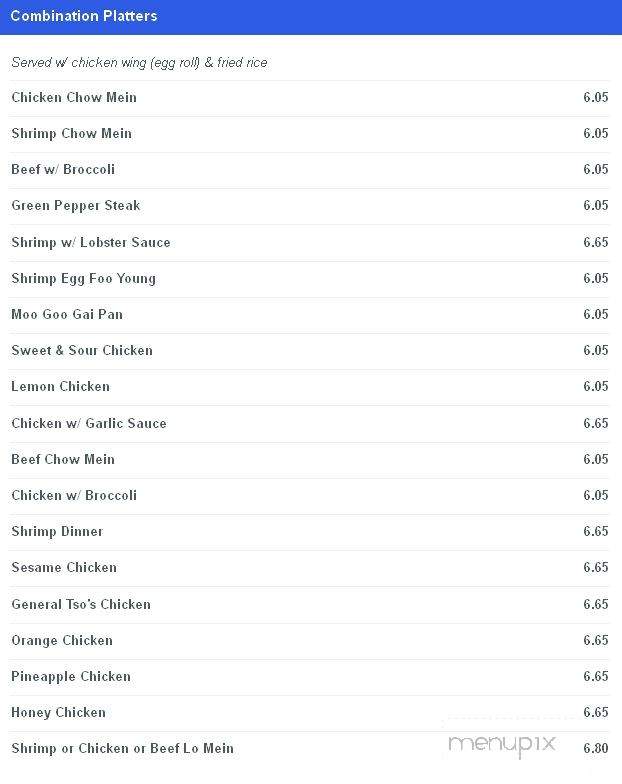This is a detailed screenshot of a restaurant's menu, focusing on the Combination Platters section. At the top, there is a blue header featuring white text on the top left reading "Combination Platters." Just below, a white header with gray highlighted text states, "Served with Chicken Wing, Egg Roll, and Fried Rice." The menu items are listed beneath this header, each demarcated by thin gray lines above and below. 

Listed from top to bottom, the menu items include:
1. Chicken Chow Mein - $6.05
2. Shrimp Chow Mein - $6.05
3. Beef with Broccoli - $6.05
4. Green Pepper Steak - $6.05
5. Shrimp with Lobster Sauce - $6.65
6. Shrimp Egg Foo Young - $6.05
7. Mugu Gai Pan - $6.05
8. Sweet and Sour Chicken - $6.05
9. Lemon Chicken - $6.05
10. Chicken with Garlic Sauce - $6.65
11. Beef Chow Mein - $6.05
12. Chicken with Broccoli - $6.05
13. Shrimp Dinner - $6.65
14. Sesame Chicken - $6.65
15. General Tso's Chicken - $6.65
16. Orange Chicken - $6.65
17. Pineapple Chicken - $6.65
18. Honey Chicken - $6.65
19. Shrimp, Chicken, or Beef Lo Mein - $6.80

Adjacent to the final price, there is a subtle watermark across the menu with grainy gray text saying "menu picks" in lowercase sans serif font, enclosed by a very faint, blocky thin gray outline.